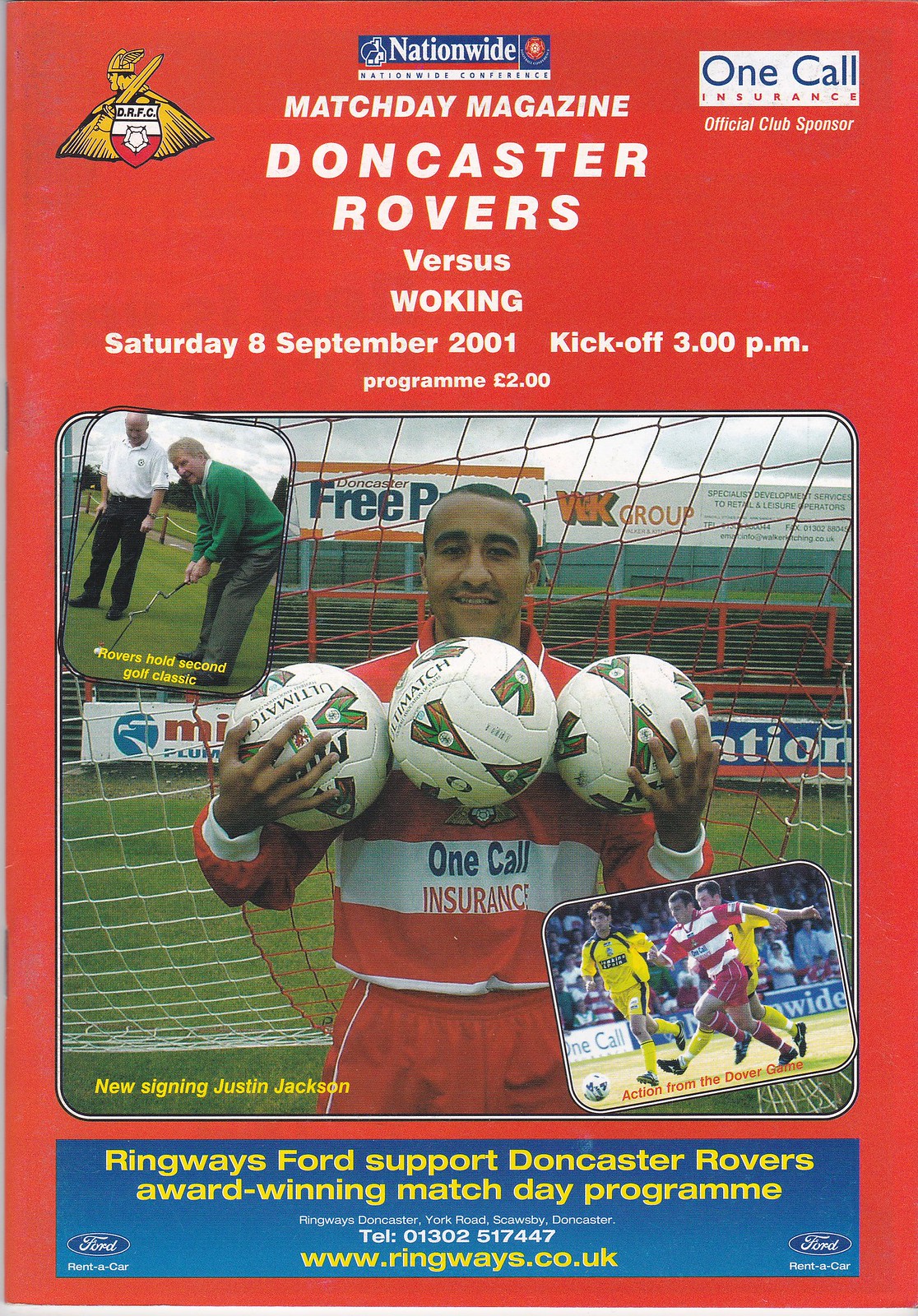The cover of the Nationwide Matchday Magazine dated Saturday, September 8, 2001, features Doncaster Rovers vs. Woking with a kickoff at 3 p.m., priced at two pounds. Prominently displayed is Doncaster Rovers' new signing, Justin Jackson, in a red and white striped jersey adorned with the One Call Insurance logo. Jackson is captured holding three soccer balls, each in a hand and the middle one in front of his chest, with a smile on his face while standing in front of the goal net. The background is red with white text, highlighting various notable contents such as "Rovers Hold Second Golf Classic" with an accompanying image of men golfing, and "Action from Dover Game." At the bottom, it details Ringways Ford’s support for Doncaster Rovers' award-winning matchday program, displaying the Ford logo in the bottom corners. Contact information for Ringways, including their Doncaster, York Road, Scosby address, phone number (013-02-517-447), and website (www.ringways.co.uk), is provided, along with a "rent a car" advert. The football club's logo is also positioned at the top.